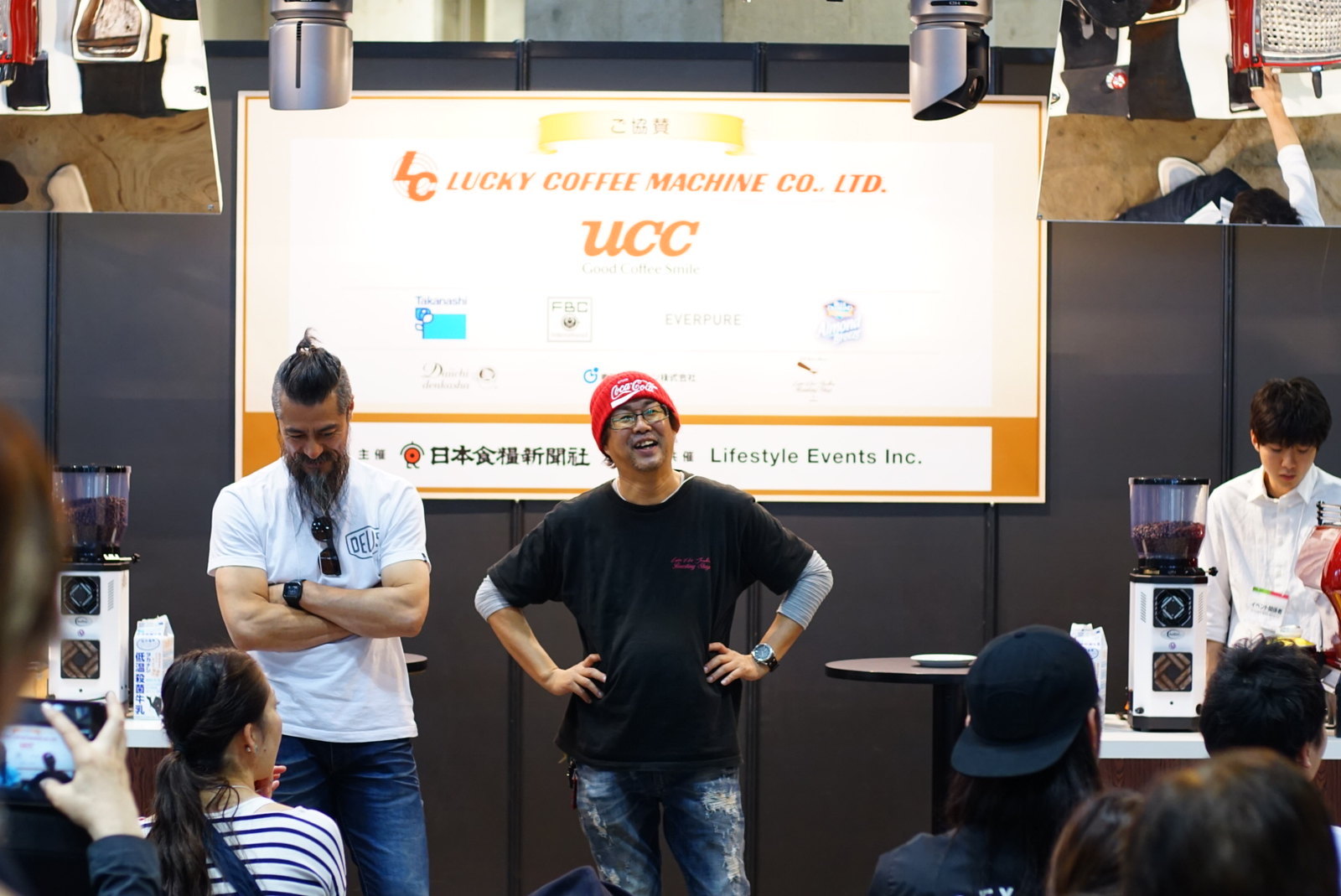At a corporate event for Lucky Coffee Machine, LTD, two men stand at the front of a conference room giving a presentation. A large screen behind them displays the company's name, UCC, and Lifestyle Events, Inc., accompanied by images and Asian writing. The man on the right, dressed in a red Coca-Cola hat and a black T-shirt, smiles and engages with the audience. Beside him stands another man in a white T-shirt with a long beard, who looks down as if focused on his task. Flanking them are coffee grinders, and mirrors are strategically placed above to demonstrate the grinding process to the seated crowd. The room features two cameras at the top, likely projecting close-up views onto the screen for better visibility. Most attendees appear to be of Asian descent, reinforcing the event's cultural context.